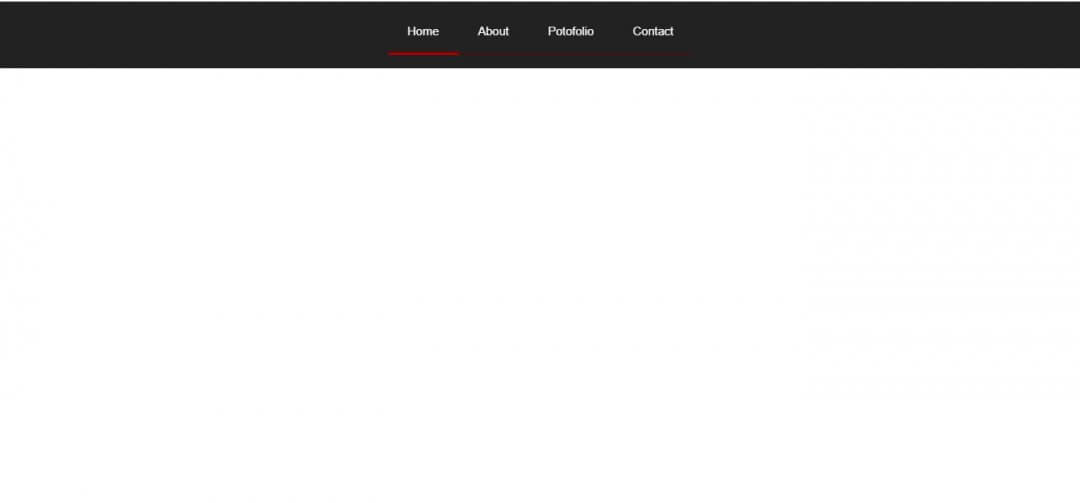The image features a minimalist black navigation bar, prominently displayed against a plain backdrop, presumably atop a website's homepage. The navigation bar, rendered as a black rectangular strip, is adorned with white text, listing four menu options: Home, About, Portfolio, and Contact. The "Home" option is distinctly emphasized with a red underline, indicating the current active page. Other than this header, the remainder of the page is notably blank, offering no further visual or textual content. This navigation bar encapsulates a standard website layout where "Home" provides an overview, "About" details the business's origins and purpose, "Portfolio" showcases work samples or projects, and "Contact" offers communication options such as phone, email, and social media handles.